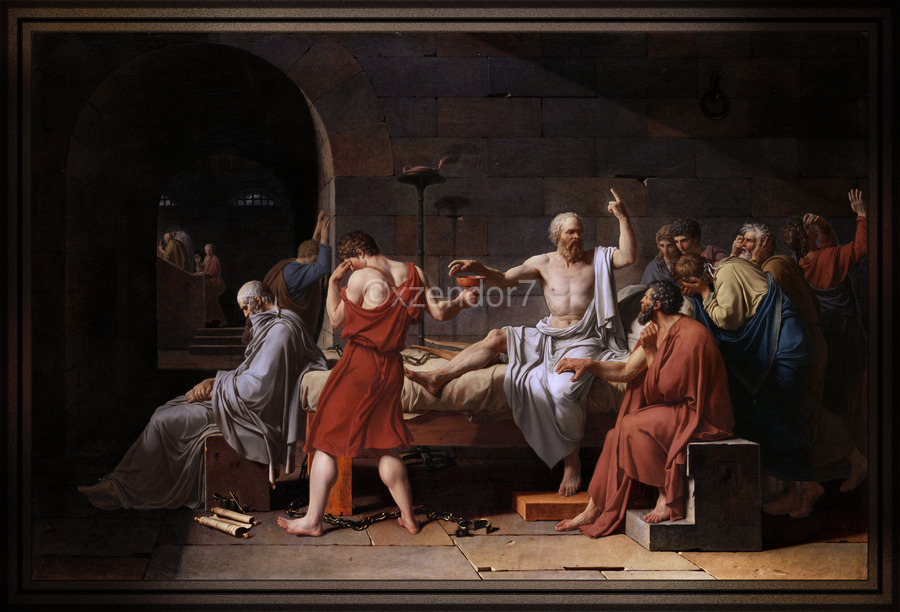The painting is a detailed depiction of a profound and somber scene, characterized by an assembly of nine to ten men clad in ancient Roman togas of varying colors—red, blue, white, and brown—gathered in a somber indoor setting that could be a stone building or a dungeon. Central to the composition is a single-person bed where a prominent man with gray hair and beard sits, partially unclothed, holding a bowl and extending his left hand upwards with his index finger pointed toward the ceiling, exuding an aura of authority and earnestness. Surrounding him, the men appear emotionally distressed; one holds his head in his hands, another seems to cry with his head bowed, and a third sits in a chair at the forefront, looking utterly dejected. Notable details include leg chains lying unattached by the bed's front leg and a musical instrument placed on the bed. The background is shadowy, enhancing the painting’s grave and reflective tone. Moreover, a watermark reading "X copyright X Z E N D O R 7" is centrally placed in a faded white font, subtly marking the piece. This image is reminiscent of the event of Socrates' final moments as he prepares to ingest poison, a significant narrative from ancient philosophy, reflecting themes of resignation, contemplation, and the stark reality of impending death.